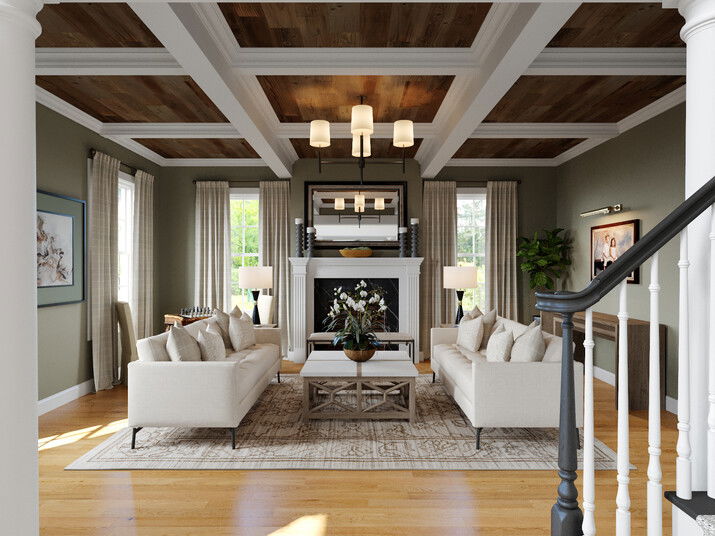This rectangular, landscape image depicts an elegant and spacious living room with a blend of traditional and modern decor elements. Central to the scene are two white couches, each adorned with several pillows, facing each other with a white tabletop with wooden legs placed in between them. A cream-colored, patterned area rug anchors this seating arrangement, resting atop light-colored hardwood floors.

The upper portion of the image features a striking wooden ceiling complemented by white beams that crisscross for added visual interest. Hanging from the ceiling is a contemporary light fixture with four yellow-glowing lampshades that illuminate the room warmly.

At the center of the back wall stands a white fireplace, topped with a mirror and flanked by decorative candles and a bowl on its mantel. Nearby, a green plant adds a touch of nature to the setting. The walls are painted in a soft gray, which harmonizes beautifully with the long, cream-colored curtains that frame three windows, allowing natural light to flood the room.

On the right side of the image, a staircase with black handrails and white spindles leads the eye upward, accentuated by a prominent white pillar. Artworks and photographs, including a picture of children and an artistic drawing, adorn both side walls, adding personal and artistic touches to the space.

Overall, this room exudes a sense of warmth and sophistication, characterized by its neutral color palette, wooden textures, and elegant furnishings.